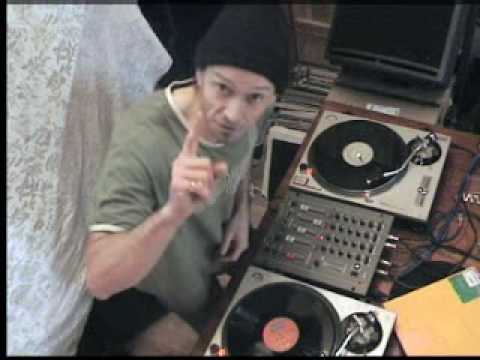This detailed, overhead color photograph captures a DJ at his table, possibly from the 50s or 60s, given the attire and equipment style. The DJ, a white, beardless man, wears a black beanie and a light green shirt with white trim around the collar and sleeves. He looks up at the camera with a serious expression, his right arm bent at the elbow and his index finger pointed upward, perhaps in mid-gesture. The tabletop features a central gray soundboard bristling with various buttons and sliders, flanked by two turntables, each spinning an album. A brown manila envelope rests in front of the setup, while chords snake around the equipment, and a speaker is positioned beside the left turntable. Behind the DJ hangs a white lace fabric, adding a contrasting texture to the scene.